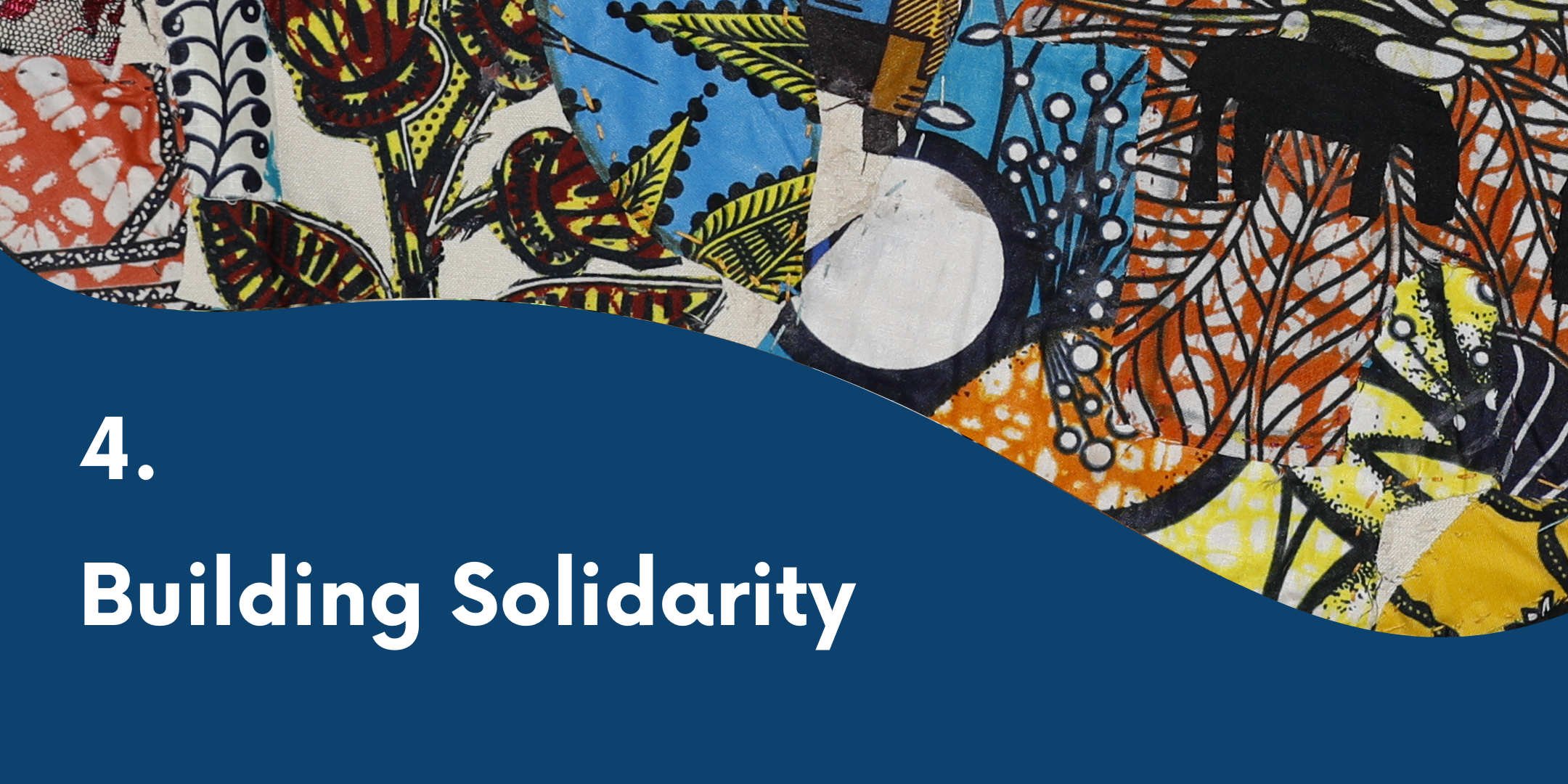The image is a computer-generated, rectangular design, approximately five to six inches wide and three inches high, possibly part of a book header or footer. At the top, a vibrant collage of different patterns and colors extends from left to right. This collage features an array of flowers and plants depicted in a variety of colors: red, white, dark burgundy, yellow, blue, orange, and burnt orange. The design displays geometric shapes including black branches, brown and yellow leaves, and blue fields, with more intricate details such as white circles bordered in black and patterns resembling leaves. In the lower left quadrant, within a dark blue background that sweeps upward and outwards in a wave-like shape, the number four is prominently displayed in white, followed by "Building Solidarity" in large white letters. The diverse and colorful top half contrasts with the solid blue bottom portion, creating a visually engaging composition that suggests an introductory slide for a presentation.